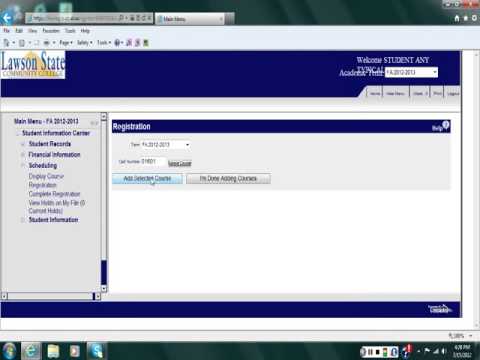Screenshot of a community college website displayed on an older Windows XP operating system. The web browser used is confirmed to be Internet Explorer, evidenced by its selection in the taskbar, alongside an open Spotify application. The web page in focus features a blue top navigation bar displaying the text "Lawson State Community College" coupled with a triangular logo reminiscent of a Triforce symbol. Towards the right, the text "Welcome to Any Typical Academy" is partially visible, highlighting significant overlap errors in the website's design. 

Below the main navigation bar, a raised gray submenu provides various menu options, albeit too blurry to read. The left side of the page presents a separated menu with blue buttons, suggesting hyperlinked tabs, showcasing the web design typical of the early 2000s, specifically around 2001. The primary section of the page is marked "Registration" in white text against a blue background, though the details of the content below remain indiscernible. The overall aesthetic, functionality issues, and design elements indicate the age and technological context of the webpage.